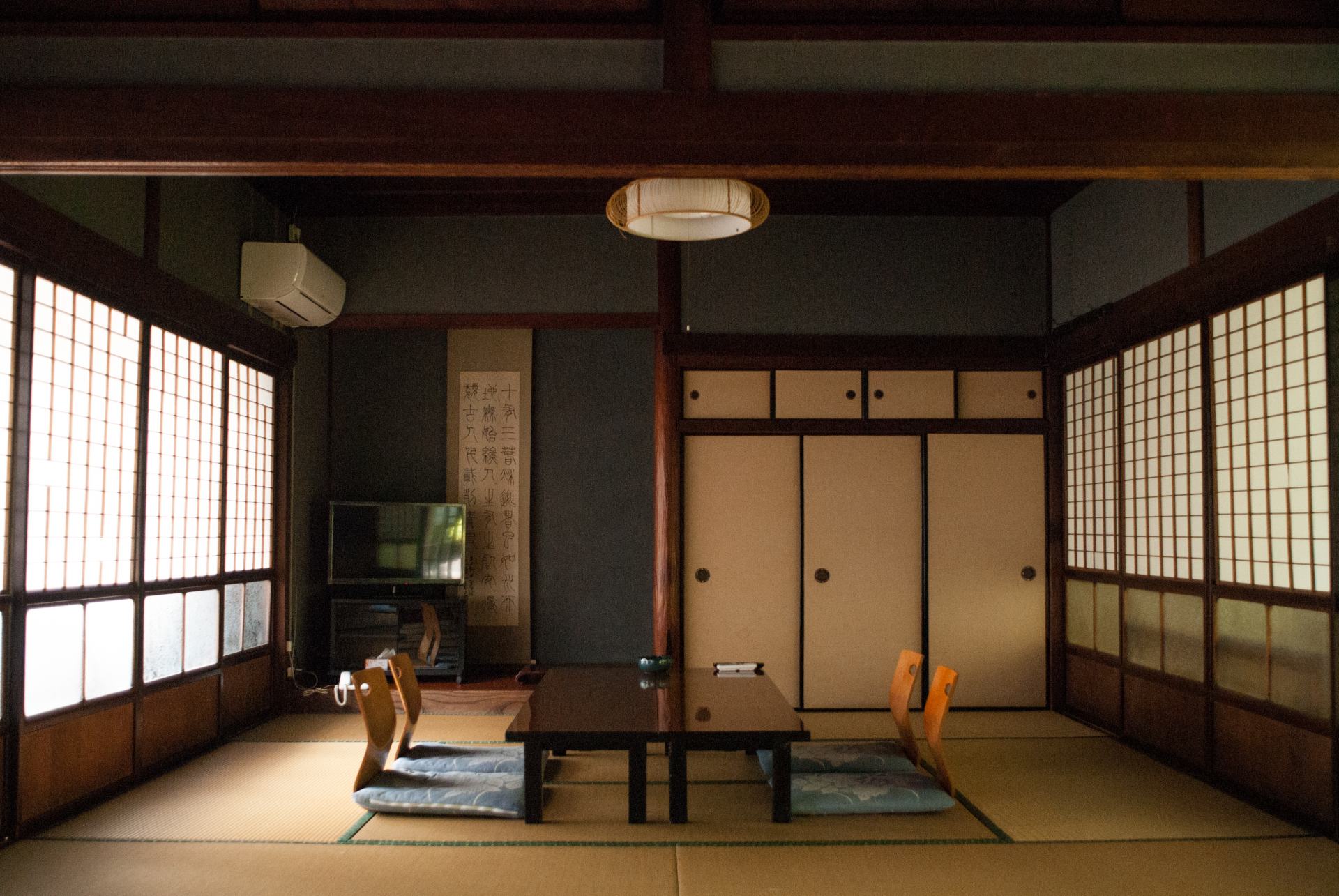This horizontal rectangular image depicts a long, narrow room with a distinctly Japanese style. The dimly lit room is adorned with slate blue walls outlined in dark wood, contributing to its serene ambiance. Both sides of the room feature windows divided into small squares by vertical and horizontal brown lines, allowing only limited light to filter through. A dark wood table sits at the center, flanked by four legless chairs in traditional Japanese style, each with a light blue cushion patterned in white designs. The chairs have differently colored wooden backs: the left pair brown, the right pair orange.

On the right side, a storage area features a set of three light wood panel doors with dark brown knobs at the bottom, and four smaller cabinets above. Adjacent to this, another set of intricately divided windows mirrors those on the left. Adding to the room's structural elegance, wooden beams stretch across the ceiling, enhancing the room's subdued palette of dark and light grays. At the far end of the room, a large flat screen TV sits unobtrusively on a stand, completing the space's harmonious blend of traditional and modern elements.